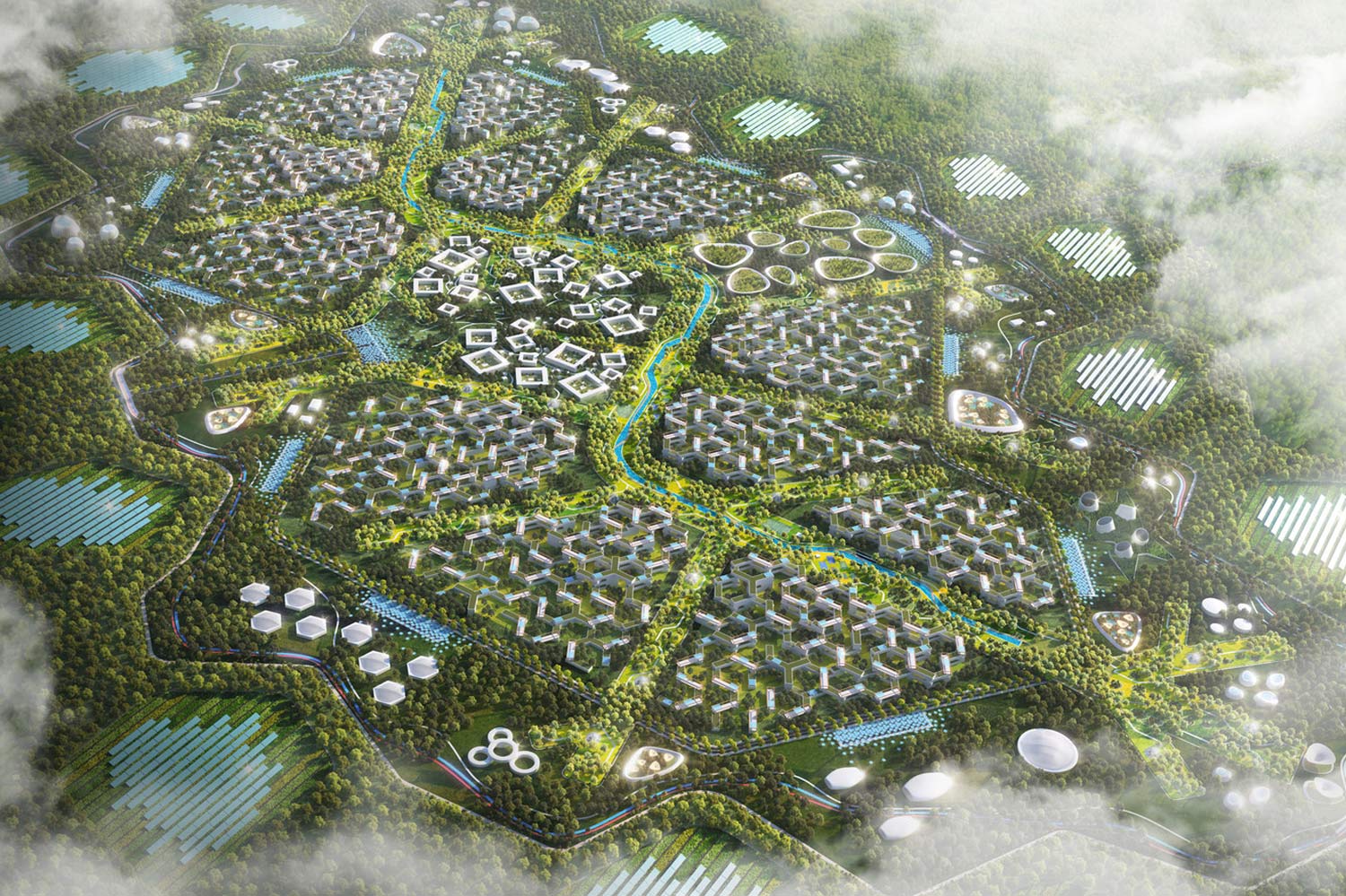This aerial image provides a detailed bird's-eye view of a unique landscape characterized by a mix of natural and man-made elements. The scene is dominated by a vast expanse of greenery, punctuated by a river or stream snaking through the middle. To the right, the sky is crowded with clouds and fog, creating a stark contrast against the relatively clearer left side. Scattered throughout the image are numerous geometric shapes, including squares and circles, which appear to be various buildings or structures. Notably, the bottom left corner features eight circular buildings. Surrounding the main area, shiny blue panel fields create a distinctive border, somewhat resembling solar panels or reflective surfaces. A series of large, pole-like objects are also distributed around the edges, adding to the sense of organized, yet enigmatic, design. There are no visible roads or vehicles, leaving the exact purpose and scale of this complex open to interpretation.